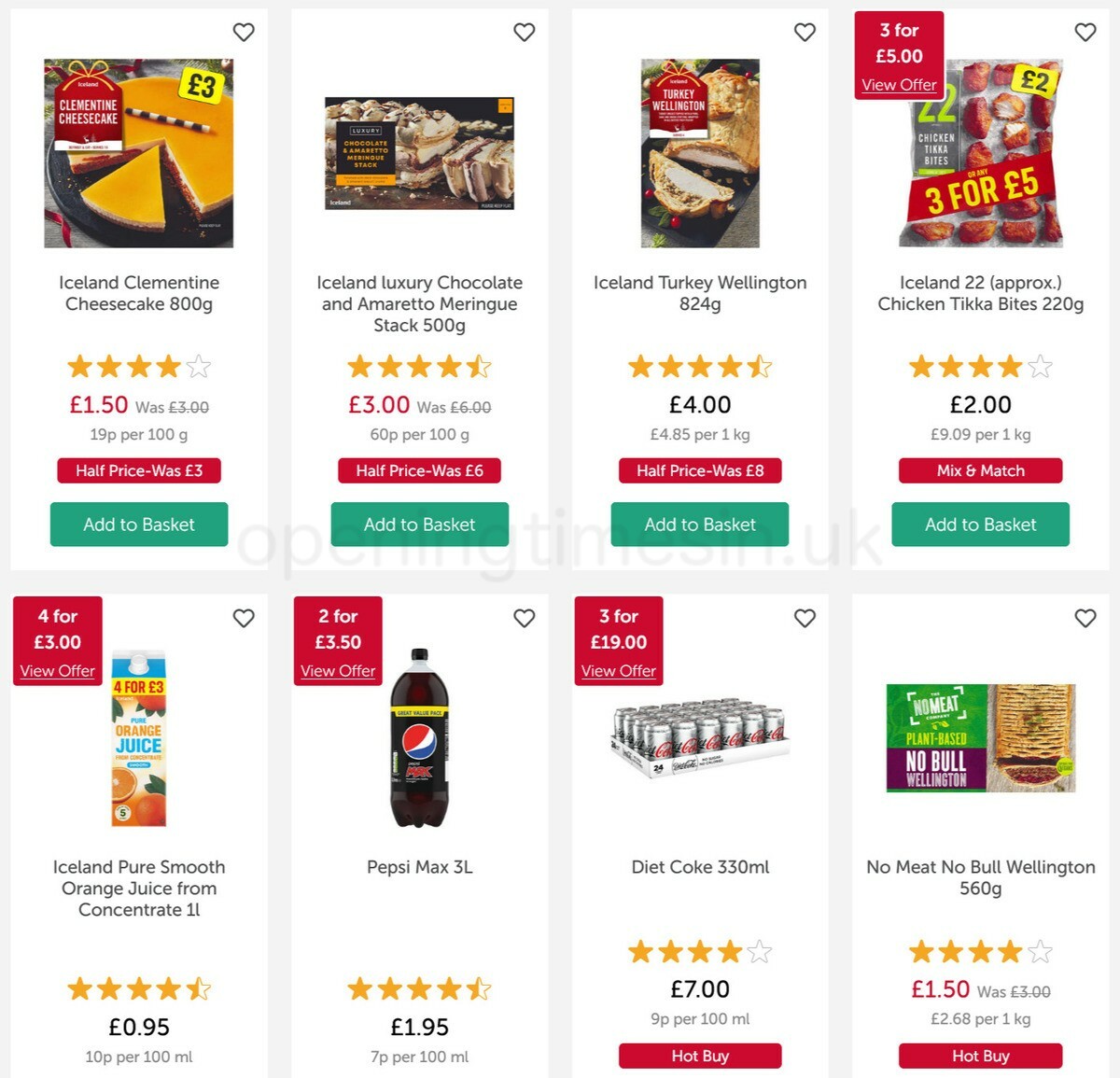The image features a light purple background with eight neatly arranged product boxes. Each box is accented with a black heart in the upper right corner. Below is a detailed description of each product:

1. **Iceland Clementine Cheesecake**
   - Rating: ★★★★☆
   - Price: $1.50 (originally $3.00, now at half price in red)
   - Button: Green "Add to Basket"

2. **Iceland Luxury Chocolate & Amaretto Meringue Stack (500g)**
   - Rating: ★★★★½
   - Price: $3.00 (half price indicated in red)
   - Button: Green "Add to Basket"

3. **Iceland Turkey Wellington**
   - Rating: ★★★★½
   - Price: $4.00 (half price indicated in red)
   - Button: Green "Add to Basket"

4. **Iceland Approximately 22 Chicken Tikka Bites**
   - Rating: ★★★★☆
   - Price: $2.00 (mix and match offer highlighted in red)
   - Button: Green "Add to Basket"

5. **Iceland Pure Smooth Orange Juice from Concentrate**
   - Note: "4 for $3.00" in the upper left corner
   - Rating: ★★★★½
   - Price: $0.95

6. **Pepsi Max (3L)**
   - Promo: "2 for $3.50" in a red box
   - Rating: ★★★★½
   - Price: $1.95

7. **Diet Coke (Case)**
   - Promo: "3 for $19.00 - View Offer" in a red box
   - Rating: ★★★★☆
   - Price: $7.00 (hot buy offer in red)

8. **No Meat Bull Wellington**
   - Rating: ★★★★☆
   - Price: $1.50 (hot buy offer in red)